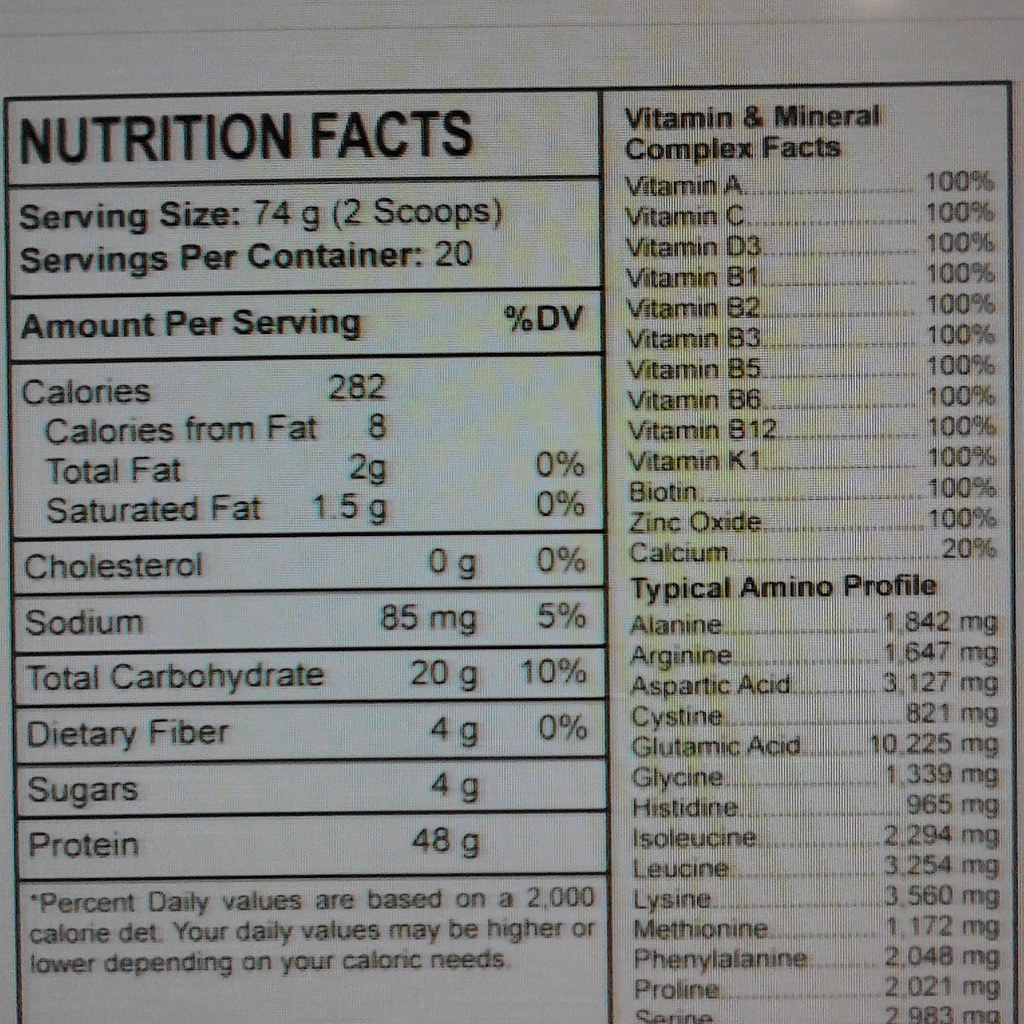The product in the image is a nutritional supplement intended to be mixed into a shake. The serving size specified is 74 grams, which equates to two scoops. Each container provides 20 servings, with each serving containing 282 calories, including 8 calories from fat. The fat content per serving is 2 grams, with 1.5 grams being saturated fat. The supplement contains no cholesterol, 85 milligrams of sodium, and 20 grams of carbohydrates.

On the right side of the product label, there is a detailed list of vitamin content, all of which are provided at 100% of the recommended daily value, including vitamins and other essential nutrients such as biotin and zinc oxide. Additionally, the label states that one serving provides 20% of the daily calcium requirement.

Furthermore, the label includes an alphabetical list detailing the typical amino acid profile found in the protein content of the supplement. Each amino acid's quantity is listed in milligrams.